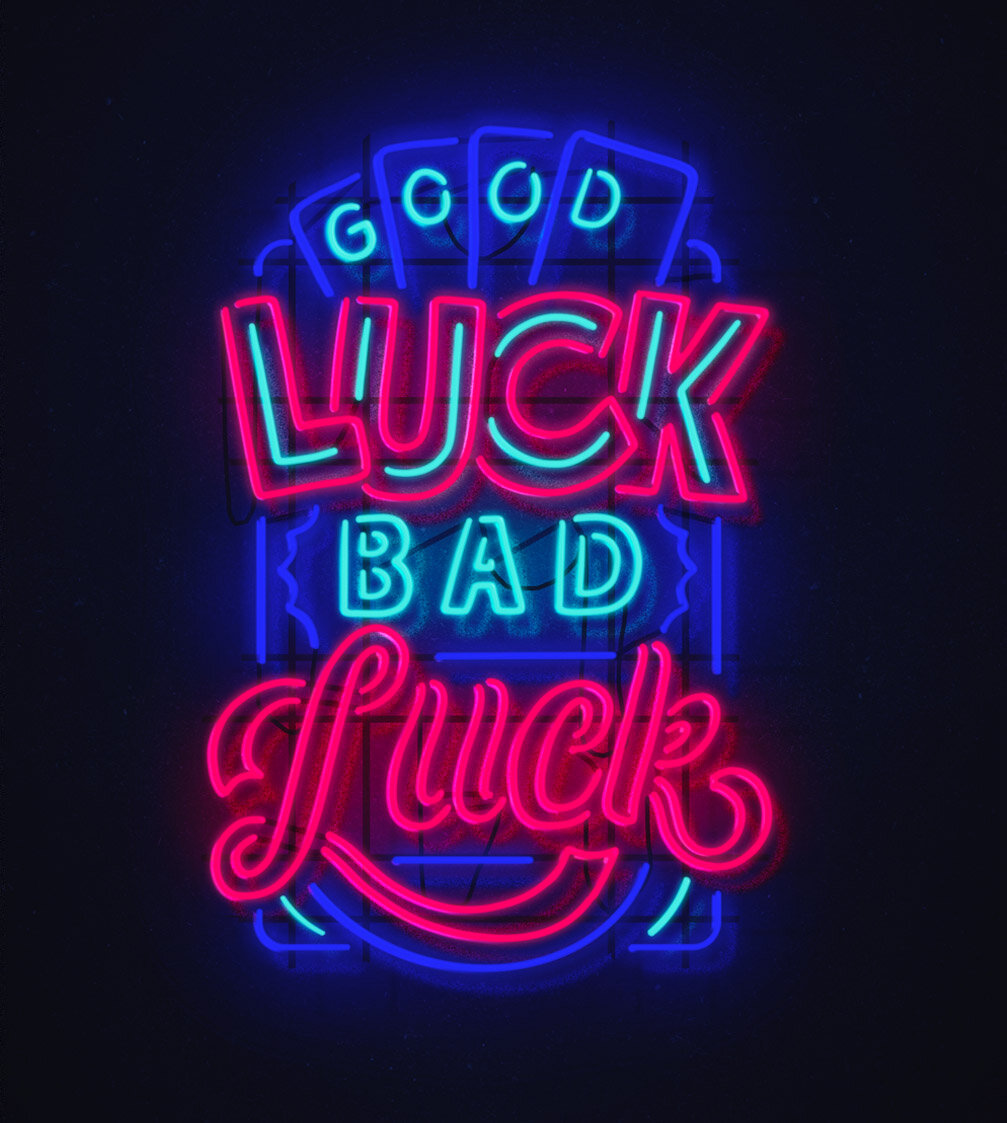The image features a neon sign which appears to be indoors, possibly in a dimly lit room or a casino-like setting. The sign itself is the sole source of light within the dark room, creating a stark contrast against the surrounding shadows. The neon sign displays the phrase "Good Luck, Bad Luck." The words "Good" and "Bad" are illuminated in a light blue color, while the word "Luck" is shown in a red hue. There is a distinctive design difference between the two instances of "Luck." The upper "Luck" is in a standard typeface with light blue lights accenting each letter, whereas the bottom "Luck" is written in a cursive font. Each word in the sign is placed within individual frames resembling cards, enhancing the casino-themed aesthetic of the image. The rest of the neon sign is predominantly dark blue, adding to the overall moody and atmospheric feel.